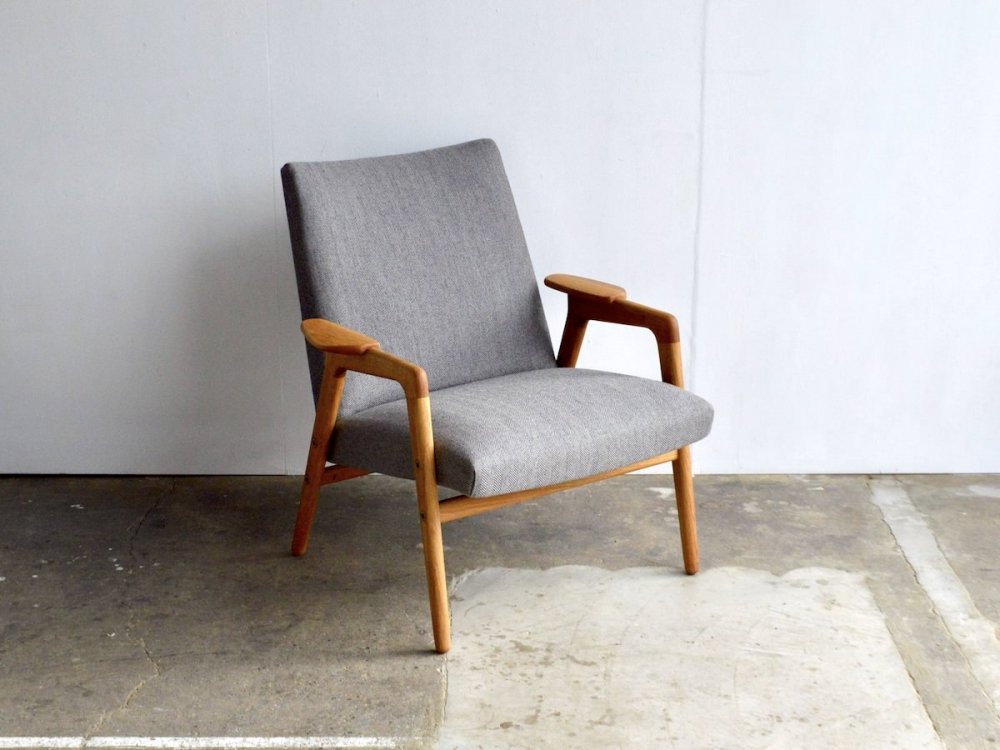The image features a solitary gray mid-century modern chair, distinguished by its gray fabric upholstery and wooden armrests, legs, and support bars. The chair is placed indoors, centered on a concrete floor with subtle color variations beneath it. Positioned at a slight diagonal, it rests near a light gray wall that features a visible seam in its right third section. The surroundings suggest a minimalistic setting, likely within an industrial or warehouse-like space, devoid of any text or additional objects. The colors in the image encompass shades of gray, brown, light gray, white, and tan, contributing to the stark, understated atmosphere.